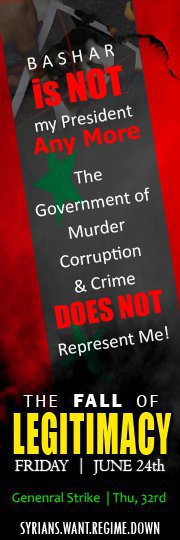This vertical advertisement poster, resembling a tall bookmark, features a vivid red and black background with a black ribbon down its center. The top of the poster boldly declares in alternating white and red letters: "Bashar is not my president anymore." Following this, the message continues in white letters: "The government of murder, corruption, and crime does not represent me!" Below this statement, it reads "The fall of" in white, with "legitimacy" prominently highlighted in large yellow letters. The bottom portion of the poster announces in white letters "Friday, June 24th" and mentions a "General Strike" marked for "Thursday, the 32nd," though likely an error for the 23rd. The concluding line states in white lettering: "Syrians want the regime down." The color palette of red, white, yellow, green, and black enhances the visual impact, making the social and political message clear and urgent.